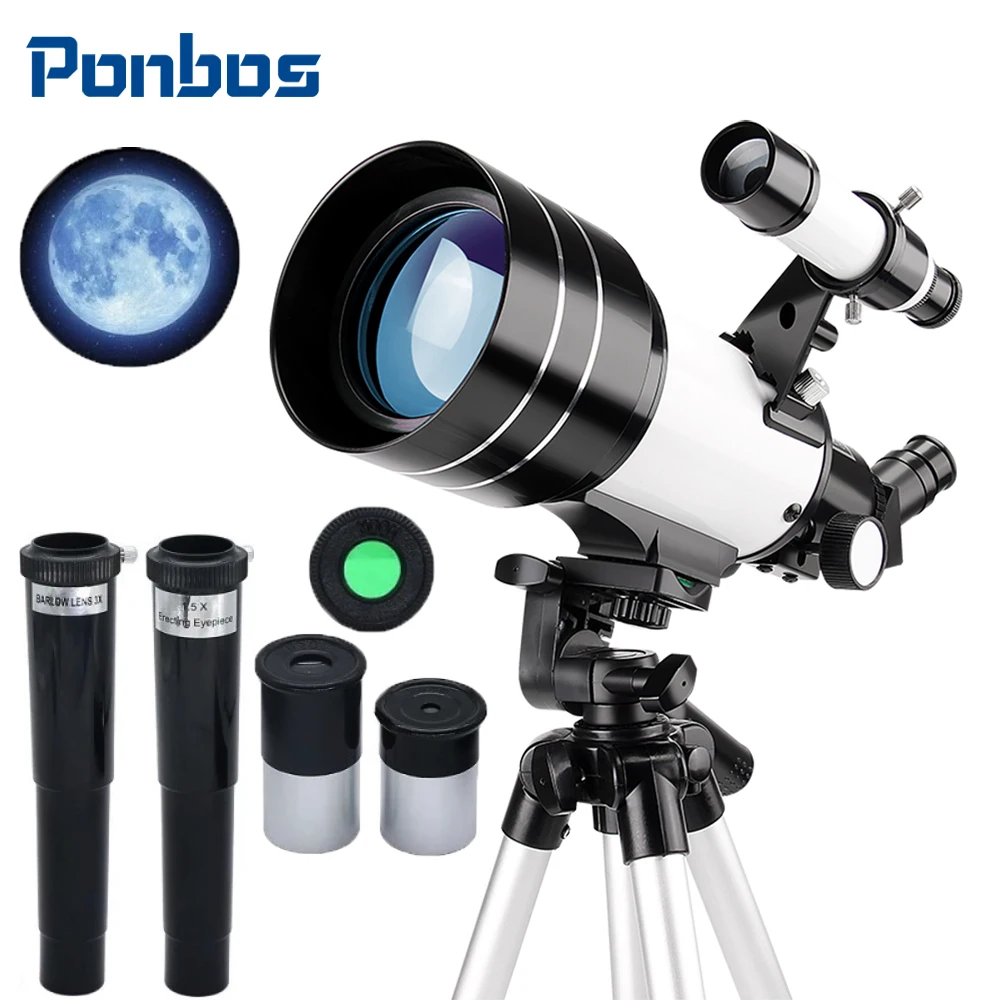This product photo showcases a PONBOS telescope prominently displayed on a white background, with every component meticulously arranged for clarity. The PONBOS brand name, styled in an intriguing blue font, is positioned at the upper left corner. Just below it, a circular inset displays a detailed image of the moon, illustrating the telescope's viewing capabilities. The telescope itself, a sleek white design with a significant open lens, is mounted on a robust tripod and oriented towards the left-hand side of the image. Surrounding the telescope are various attachments, including five interchangeable lenses, each meticulously placed to highlight its functionality. Additionally, there are other accessories like extenders and viewing gadgets, emphasizing the telescope's versatility. Despite the minimalist, photoshopped white background, the well-arranged components and the green-tinted lens piece offer a comprehensive view of this medium-grade, high-quality telescope set.